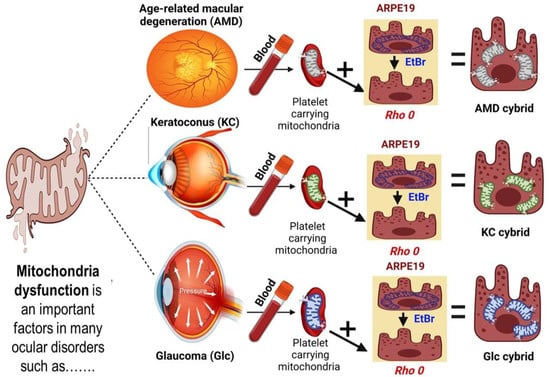The image is a detailed scientific chart, typical of those seen in medical journals or textbooks, illustrating the process of mitochondrial dysfunction and its role in several ocular disorders, presented in a flowchart format. On the far left, the chart begins with the text "Mitochondrial dysfunction is an important factor in many ocular disorders such as...," highlighting its pivotal role. Three branches extend from this text to depict specific conditions: age-related macular degeneration (AMD), keratoconus (KC), and glaucoma (GLC).

The top branch addresses age-related macular degeneration (AMD). This section includes an image of a broken mitochondrion, followed by a sequence illustrating blood, platelets carrying mitochondria, and further cellular diagrams leading to AMD Cybrid. Similarly, the middle branch illustrates the progression to keratoconus (KC), and the bottom branch details the development of glaucoma (GLC), each sequence following a comparable path involving blood components and cellular changes.

Each condition is depicted with color-coded diagrams featuring intricate details, such as the eye, blood vessels, and cellular components, in hues of dark red, orange, yellow, and touches of blue. The chart meticulously breaks down the cellular alterations and the role of mitochondria in each condition, making it a comprehensive visual representation of how mitochondrial dysfunction can lead to different ocular diseases.